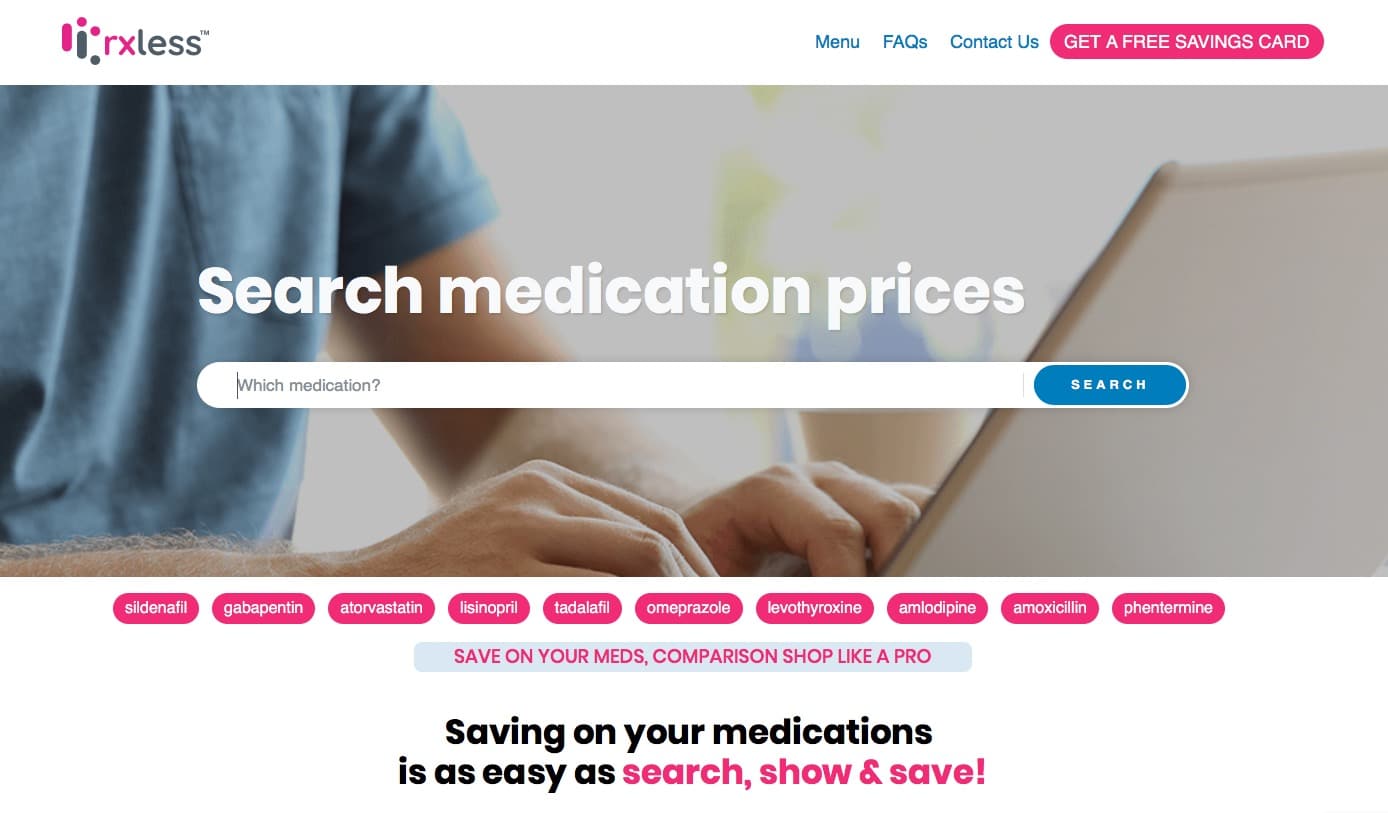In this screenshot of a website, the business's logo is prominently displayed at the top left corner. Directly to the right of the logo is a search field, where a blinking cursor is followed by the text "Which medication?". Adjacent to the search field is a blue "Search" button. Above this, a header reads "Search Medication Prices."

At the top right of the screen, there are several links including "Menu," "Frequently Asked Questions," "Contact Us," and "Get a Free Savings Card." Below these navigational elements, various names of medications are listed, such as Sildenafil, Gabapentin, and Atorvastatin.

Further down the page, text emphasizes the website's purpose with phrases like "Save on your meds," "Comparison shop like a pro," and "Saving on your medications is as easy as Search. Short and safe." The page ends with a courteous "Thank you."